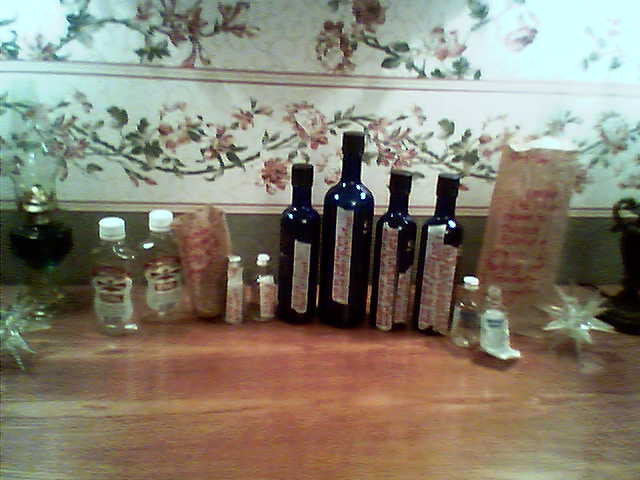This image shows various bottles neatly arranged side-by-side on a polished, light brown wooden table set against a wall adorned with horizontally striped floral wallpaper in white and green. Starting from the left, there is an old-school oil lamp, followed by two clear glass bottles with red and white labels and white caps, reminiscent of small vinegar or similar condiments. To the right of these are two extremely small glass bottles. Next are four dark, almost black, wine-like bottles with masking tape-style labels featuring red lettering. Further right, there are two more small, clear glass bottles, similar to the previous ones, and a small paper bag. The far right side of the table has another paper bag with red text, and a multi-pointed star ornament. The overall lighting in the room is dim, casting a pale blue shade, suggestive of an image likely taken in the 1980s. The photo is somewhat blurry, giving it an aged, nostalgic appearance.